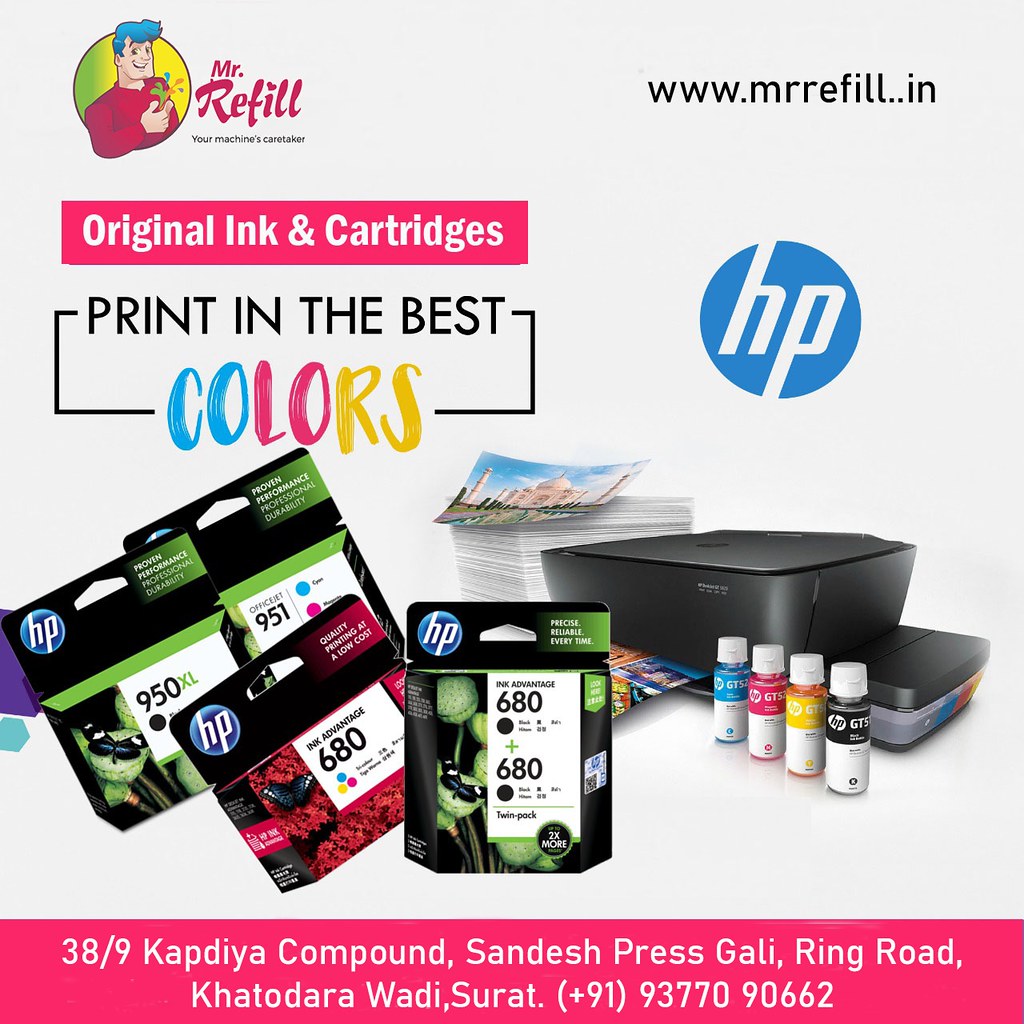The advertisement image showcases a detailed promotion for an HP printer ink refill service provided by Mr. Refill. At the top left corner, a cartoon icon of a man with blue hair and ink-splattered fingers smiles next to the caption "Mr. Refill, your machine's caretaker." The top right corner features the website address www.mrrefill.in. Down the left side of the image, a pink banner announces "Original ink and cartridges" in orange text, followed by "Print in the Best Colors" in black text, where "CO" is highlighted in blue, "LO" in pink, and "RS" in yellow. Adjacent to this is the blue and white HP logo.

Near the bottom left of the image, various boxes of printer ink are displayed, including models such as 950XL, 951, 680, and 680 Plus, with vibrant packages in green, red, and black. To the right, we see a black office printer accompanied by tubes of ink in blue, pink, yellow, and black, and a stack of printed pages. Finally, a pink banner at the image's bottom contains the address and contact number in white text: "38/9 Capdia Compound, Sandesh Press, Gali, Wing Road, Katodara, Wadi, Surat (+91 93770 90662)."